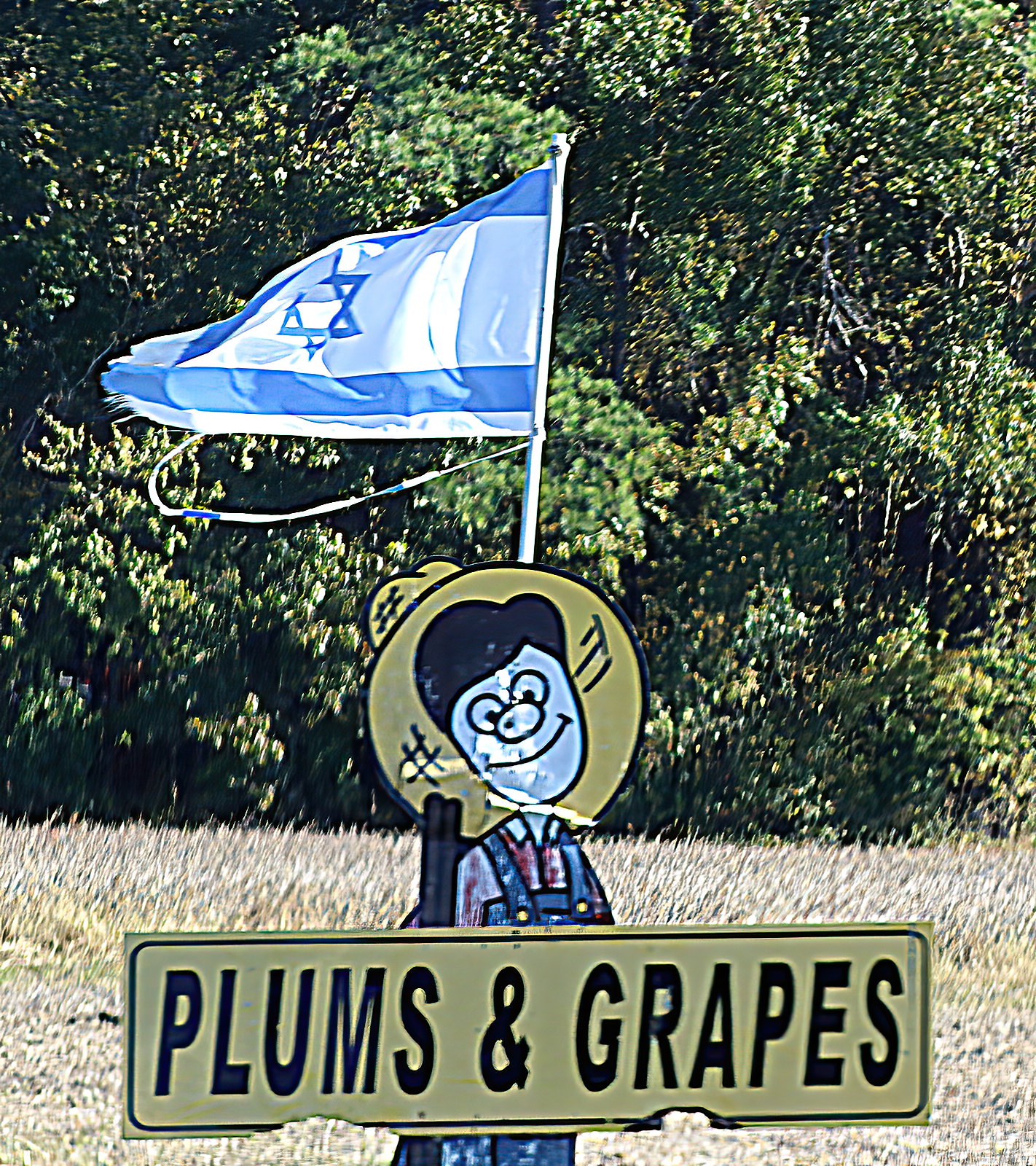The image features a central cartoon-style sign depicting a caricature of a farmer standing at the bottom of the frame. The farmer is designed with a straw hat, black hair, blue overalls, and a red shirt. He has exaggerated cartoon features, such as large eyes, a big nose, and a wide black smile. The farmer holds a bright yellow sign that reads "plums and grapes" in black text. Behind him, a blue and white Israel flag with the Star of David is visible, supported on a white pole. Surrounding the sign is a patch of yellowish grass, suggesting it might be somewhat dry. Further in the background, a dense line of trees fills the top three-quarters of the image, creating a forest-like backdrop.